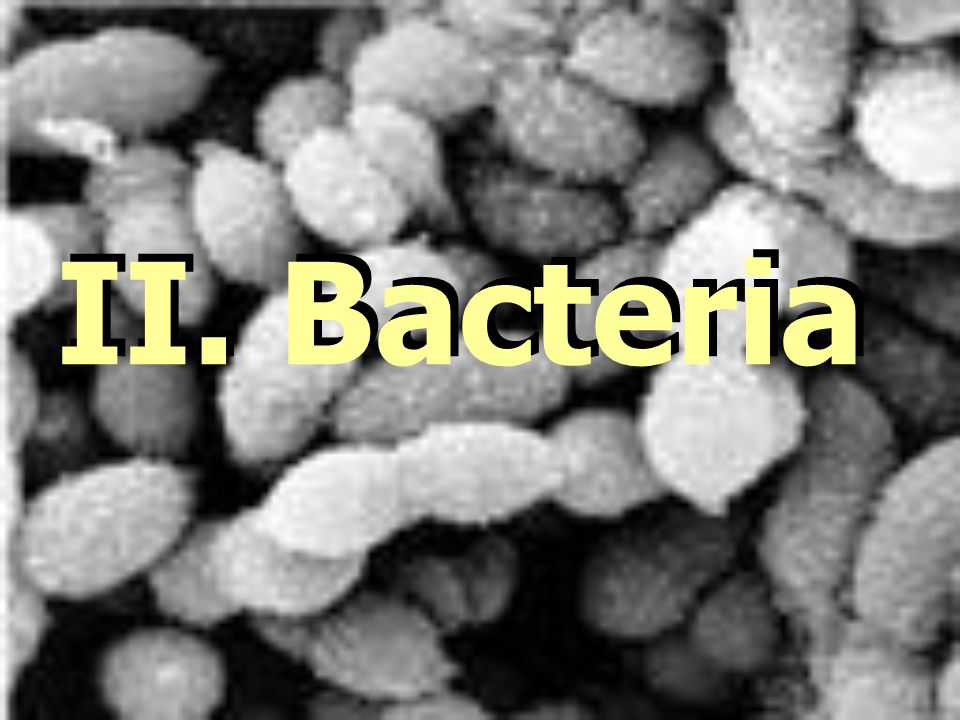This black-and-white image depicts microscopic bacteria, characterized by their round, oval, and teardrop shapes in shades of gray and white. Scattered throughout the picture, these bacteria resemble rice kernels or small pellets, highlighted against a predominantly black background, which may represent empty space or additional contrast. Central to the image is gold or pale yellow text that reads "II. bacteria," with the "II" in capital letters, a period following, and "bacteria" with a capital B. The text casts a three-dimensional shadow in black, further enhancing its presence midways across the image. The detailed depiction of bacteria combined with the striking, shadowed lettering suggests a scientific or educational focus, emphasizing the microscopic nature of the subject.